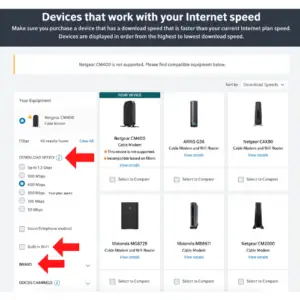Ensure that you purchase a device with a download speed that exceeds your current internet plan to avoid bottlenecks in speed. The image features a variety of tech gear, including SIM cards and several modems from multiple brands, prominently Netgear. The image showcases six modems with red arrows pointing to various download speed indicators, brand names, and specific devices. The status of different features is also marked, with one aspect circled as checked and three others identified as unchecked. The visual elements clearly highlight the importance of selecting a device that can fully utilize your internet service’s download capabilities.